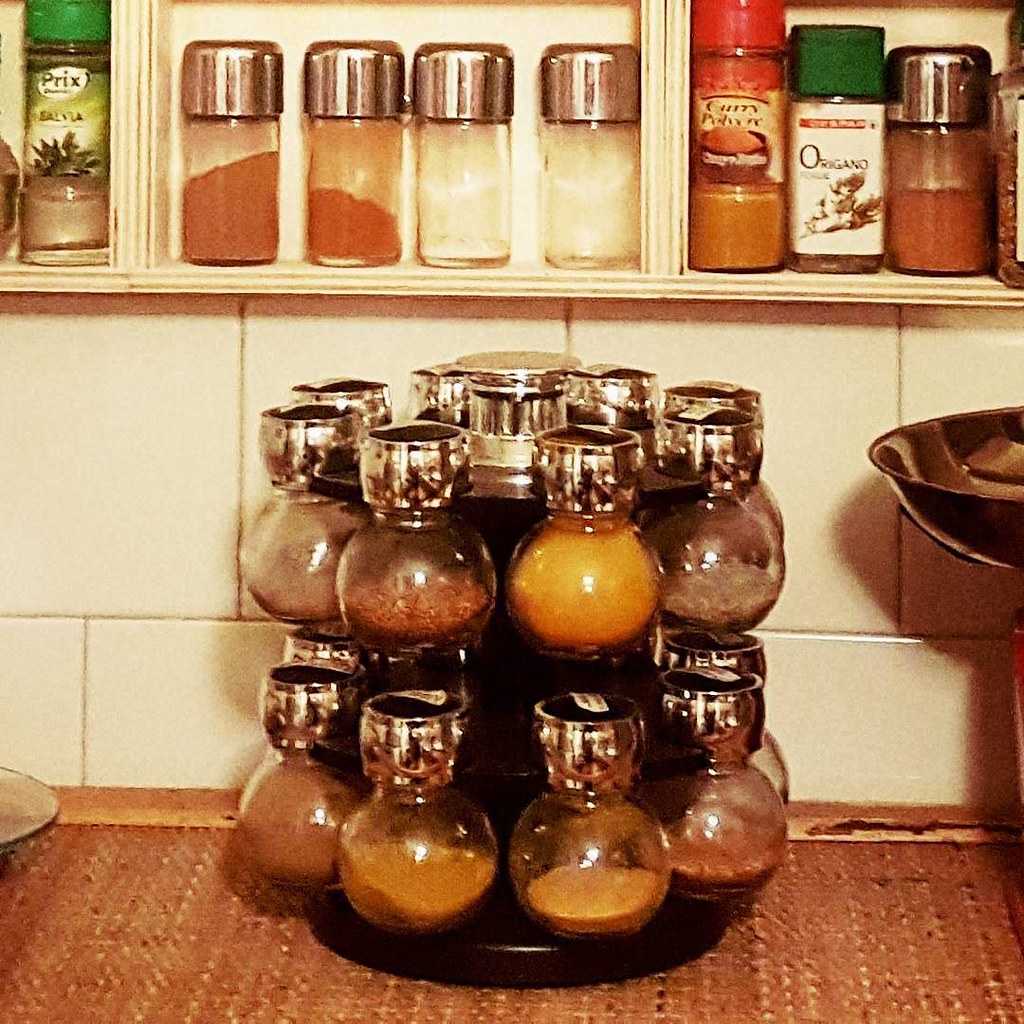The photograph depicts a detailed scene in a kitchen with a warm, yellow-orange filter. The background features a white, shallow shelf divided into three visible square sections, each holding various spice containers. The left section has a single spice bottle with a green top. The middle section contains four clear glass spice jars with metal lids; the two on the left appear to have brown spices, while the two on the right seem to contain white spices. The right section holds three spice containers, one clear glass jar with a silver lid and a brown spice, an oregano jar with a green lid, and a curry jar with a red lid.

In the foreground, sitting on a brownish countertop with a textured surface, there is a two-tiered, revolving spice rack. The rack holds several small, round spice jars with silver lids, each filled with various spices in colors ranging from yellow and brown to dark grey. Some jars are full while others are partially empty. The wall behind the countertop is adorned with green tiles and a wooden edge, adding to the kitchen's visual complexity. Additionally, the left corner of the image reveals the edge of a white plate or bowl, and the right corner shows a brown bowl resting on an unseen stand, seemingly hovering against the wall. This composition captures the organized yet eclectic nature of a well-used kitchen.